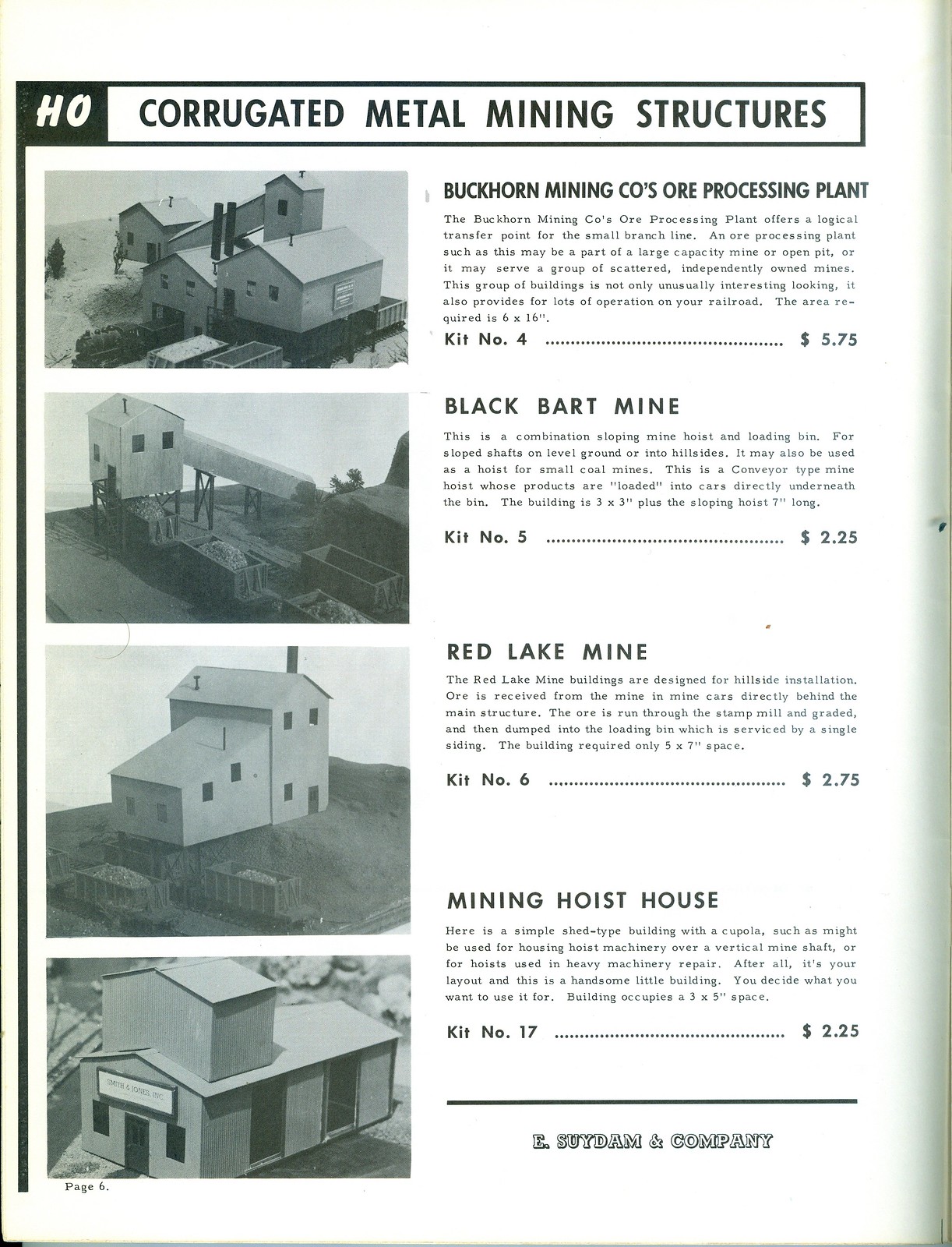This black-and-white advertisement page from an old print magazine by E. Sudam & Company features four detailed images and descriptions of various corrugated metal mining structure kits available for sale. Running vertically down the left side of the page, the images display different types of mining infrastructure that range from single-story to multi-story buildings, each designed to support the mining and ore processing activities. 

The first image is labeled "Buckhorn Mining Company Ore Processing Plant," identified as kit number 4, and is priced at $5.75. This structure consists of multiple interconnected buildings forming a comprehensive processing facility. Directly below it, the second image showcases the "Black Bart Mine," a single structure elevated on stilts with a chute extending from its front, listed as kit number 5 for $2.25. 

The third image depicts the "Red Lake Mine," a large rectangular building with a lean-to addition, possibly constructed over a body of water or trench. This is offered as kit number 6 for $2.75. Finally, the fourth image shows the "Mining Hoist House," a rectangular building with a two-story addition at one end and a peaked roof. It also features a white banner for signage above its door. This final kit is number 17, priced at $2.25.

Accompanying each image on the right side are descriptive paragraphs detailing the structures and their functionalities within mining operations. The layout ensures that potential buyers have a clear understanding of each product, complete with visual references and associated prices.